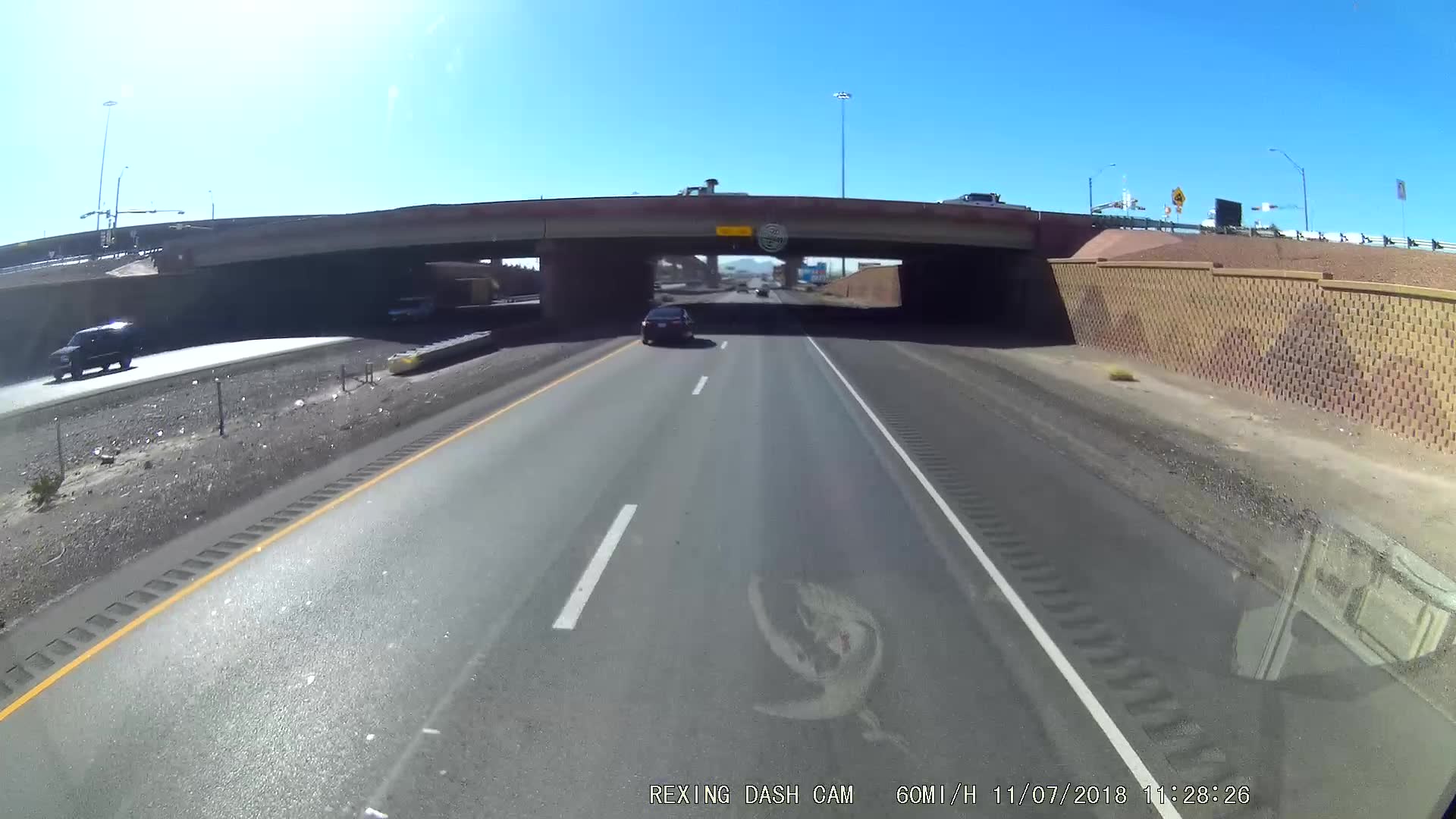This photograph, likely taken from a dashcam on a tall vehicle, captures a scene of an American highway from an elevated vantage point above the right-hand lane. The image is wide-angle, providing a broad view of the roadway ahead. Prominently in the mid-background, a bridge spans the width of the highway. In the left-hand lane ahead, another car is visible, traveling forward. To the left side of the image, one can see the oncoming traffic lane with a car moving in the opposite direction. The sky is a clear blue, extending across the top portion of the image, while a beige fence runs parallel to the road on the right side.